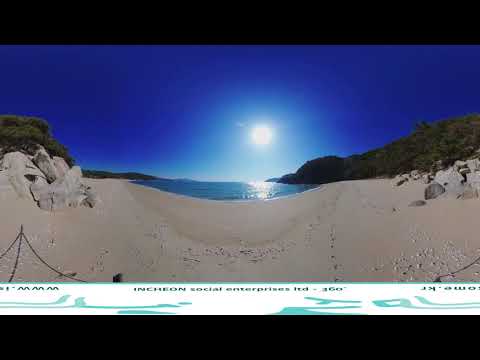The image depicts a serene beach scene under a moonlit night. At the bottom of the image, there's a sandy beach stretching across, characterized by a light tan color. The center of the image features a tranquil body of water, which brilliantly reflects the moonlight from above. The moon, with a lighter blue aura, illuminates the dark royal blue sky. To the right, there's shadowed vegetation densely covered in greenery. The entire scene has a distorted, warped perspective typical of a 360-degree lens, causing elements to bend inward at the center and curve outward at the edges. A white banner ad occupies the bottom third of the image, displaying a blue logo with the text "Incheon Social Enterprises, 360 degrees."